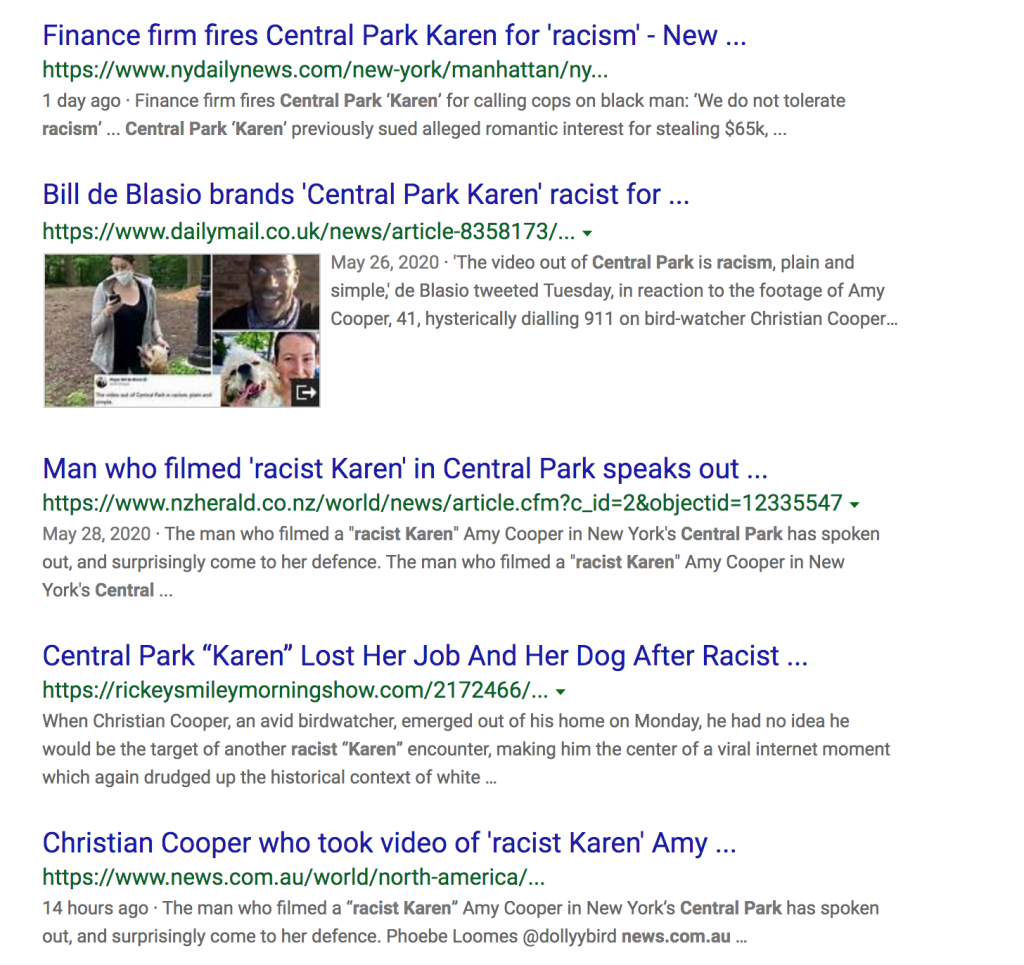**Detailed Descriptive Caption:**

The image depicts a Google search results page highlighting the aftermath of a widely publicized racist incident in Central Park, New York. The top result shows a headline from the New York Daily News: “FIRING Central Park ‘Karen’ for Racism,” dated one day ago. Below it, another headline from DailyMail.co.uk reads, “Bill de Blasio Brands Central Park ‘Karen’ Racist,” featuring an image of a woman on her phone, a black man, and another individual with a dog.

Additional search results include various articles such as:
- “Man Who Filmed Racist ‘Karen’ in Central Park Speaks Out” from the New Zealand Herald
- “Central Park ‘Karen’ Lost Her Job and Her Dog After Racist Incident” from the Rickey Smiley Morning Show
- “Christian Cooper Who Took the Video of Racist ‘Karen’ Amy” from news.com.au

These headlines reflect the extensive media coverage of a woman’s racist behavior in Central Park, with the term "Karen" used in quotations to emphasize the derogatory nature of her actions.